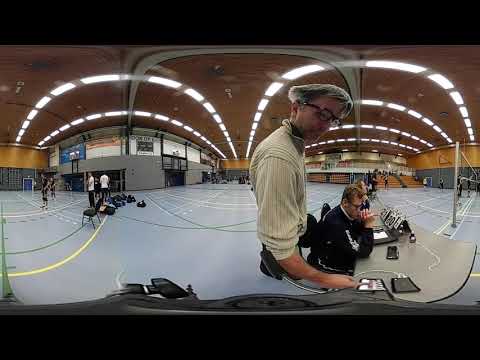The fisheye lens image captures an indoor gymnasium set up for a volleyball game. The ceiling, with its distinctive lights creating upside-down smile shapes, provides a stark backdrop to the scene. In the foreground, two scorekeepers occupy a gray counter; one with glasses and a striped pale yellow shirt is engrossed in his task, while the other, also wearing glasses but with shorter hair and a black and white striped shirt, seems focused on an electronic scoreboard. The hard, painted surface of the court is partially visible beneath the warp of the lens, and in the distance, two players stand alert by the net, ready for an imminent serve. Scattered throughout the gym, the vibrant hues of the setting include blacks, browns, grays, whites, oranges, blues, yellows, and greens, forming an eclectic canvas of an active sports event.